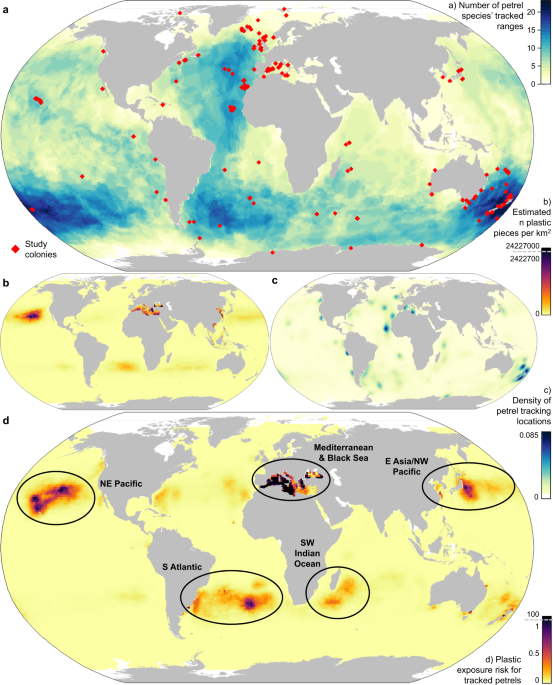The image is a vertically rectangular, multicolored composite displaying four heatmaps of the Earth, set against a white background. The largest images are situated at the top and bottom, while two smaller globes occupy the middle section. The maps use various colors such as blue, green, yellow, and red to illustrate different datasets.

1. The top heatmap highlights the number of petrel species' tracked ranges with red dots concentrated across the oceans, overlaid on grey seas and blue-green landmasses.
2. The second heatmap details the estimated number of plastic pieces per kilometer, with notable concentration in the Mediterranean Sea and portions of the Pacific Ocean.
3. The third heatmap displays the density of petrel tracking locations, represented as sparse dots scattered mainly over the oceans.
4. The bottom heatmap shows plastic exposure risk for tracked petrels, with the highest densities located in the South Atlantic, North Eastern Pacific, Mediterranean, Black Sea, and East Asia Northwestern Pacific.

A color bar on the right side indicates a gradient scale from 0 to 20, corresponding to measurements in yellow, green, blue, and black. This detailed visualization effectively communicates various environmental factors affecting petrels and plastic distribution in the world's oceans.